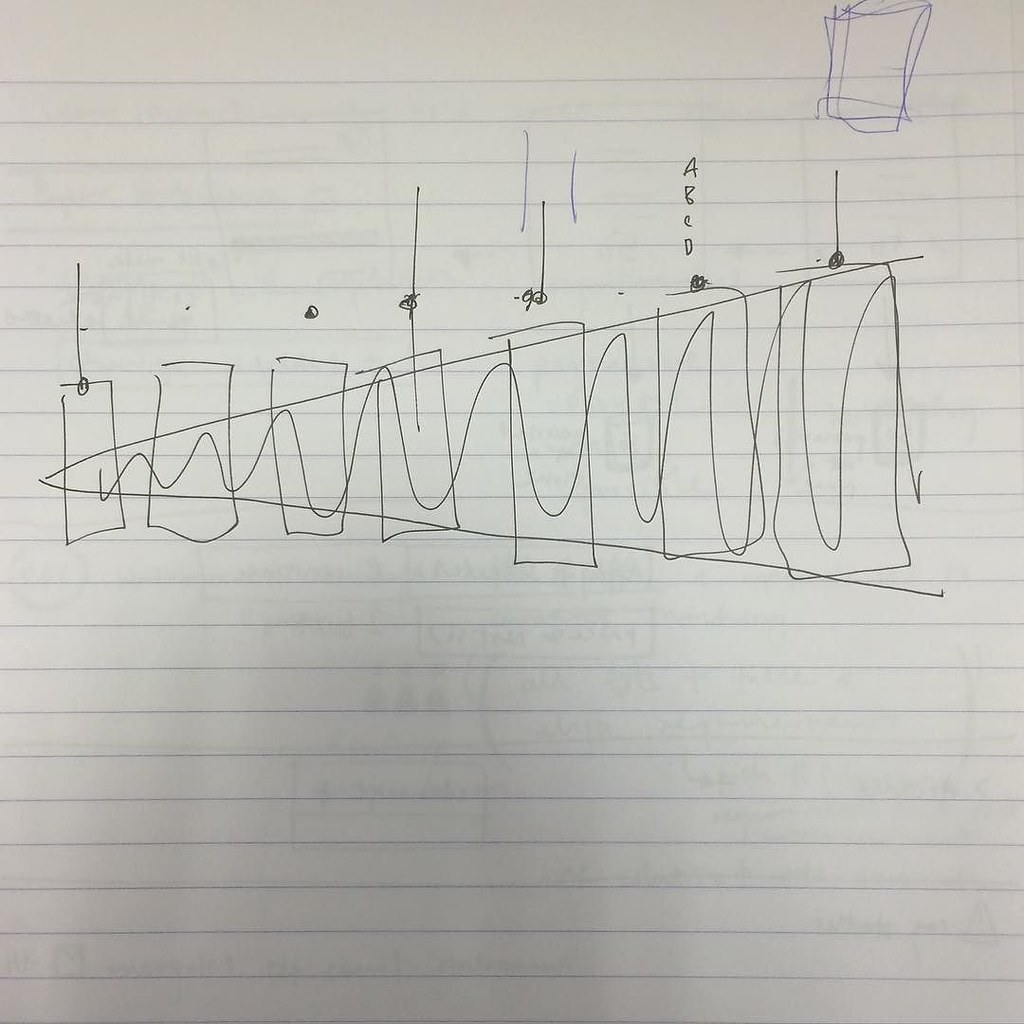A detailed sketch made with blue ink on white lined paper features a complex and somewhat chaotic mix of images and shapes. In the upper right corner, a square has been drawn multiple times over itself, creating a messy, overlapping pattern. The center of the paper is dominated by a large, left-pointing triangle that lacks a bottom side. Nested within this shape are seven rectangular forms that resemble piano keys, marked by an array of distinct symbols and lines. 

Starting from the left, the first rectangle contains a line intersecting a circle, which might resemble a musical note. The second rectangle hosts a solitary dot. The third rectangle is filled in with a solid circle. In the fourth, a line intersects a somewhat messily colored-in circle. The fifth resembles another musical note, with a line where the circle extends to the left, paired with two blue ink lines adjacent to the top of the line. In the sixth rectangle, the letters "A, B, C, D" are arranged vertically with a scribbled dot above them. The seventh contains yet another music note-like figure with a line and a black dot beneath it. 

Additionally, faint impressions from an underlying sheet of paper are visible through the current one, suggesting the presence of more sketches or writings involving squares, rectangles, lines, and dots. The overall composition of the page creates an intricate blend of musical, geometric, and abstract elements.